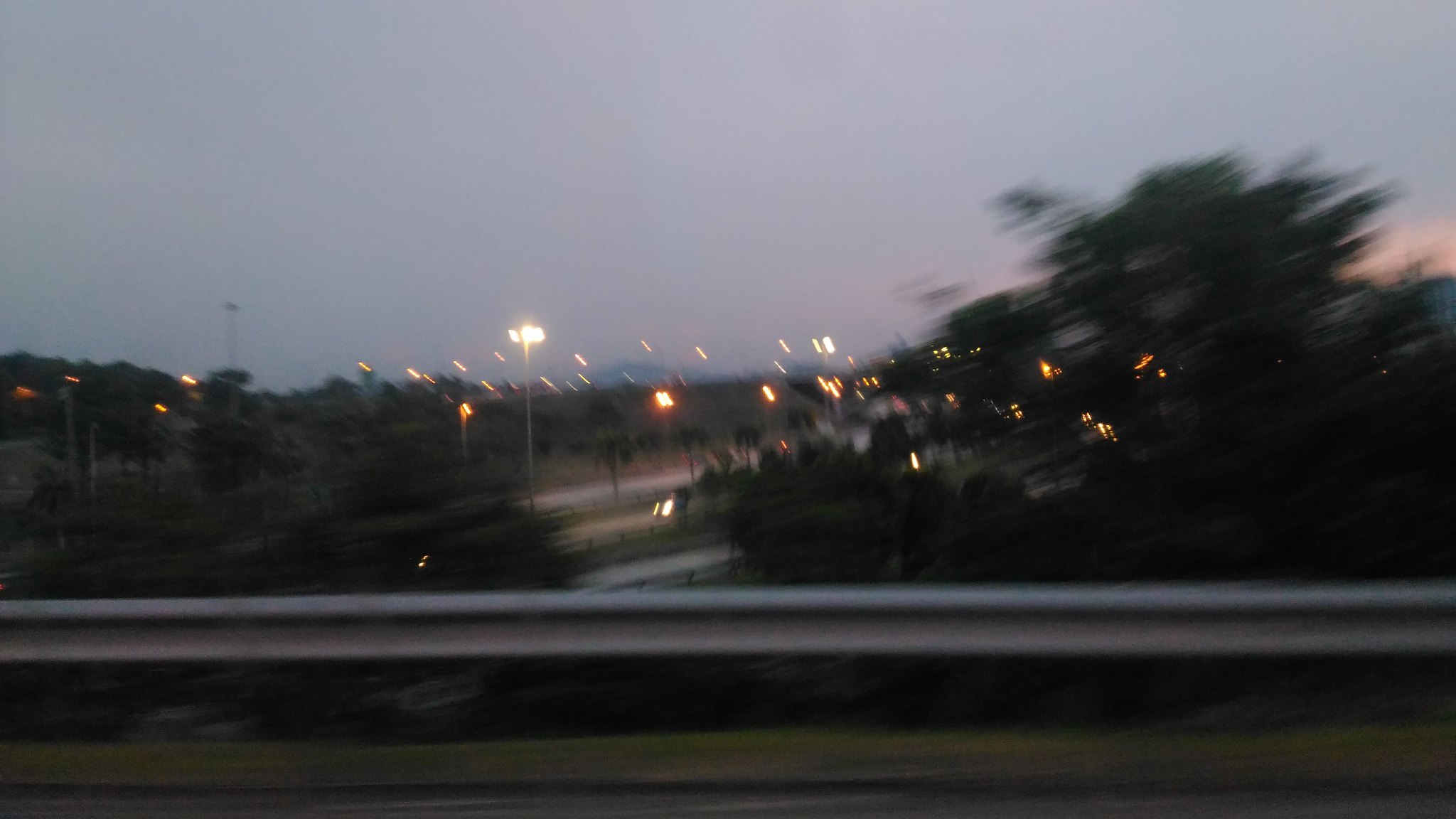Captured from a moving vehicle, this blurry nighttime photograph offers a bird's-eye view of a multi-lane highway, likely taken from an overpass. The highway below features three to four lanes, with a few cars visible navigating the roads. Streetlights, tall and bright, illuminate the scene, casting a warm glow on the asphalt below. The sky showcases a striking blend of grayish-blue hues accompanied by pink shades indicating either a setting or rising sun on the right side of the image. In the foreground, dense tree foliage partially obscures the view of the highway.